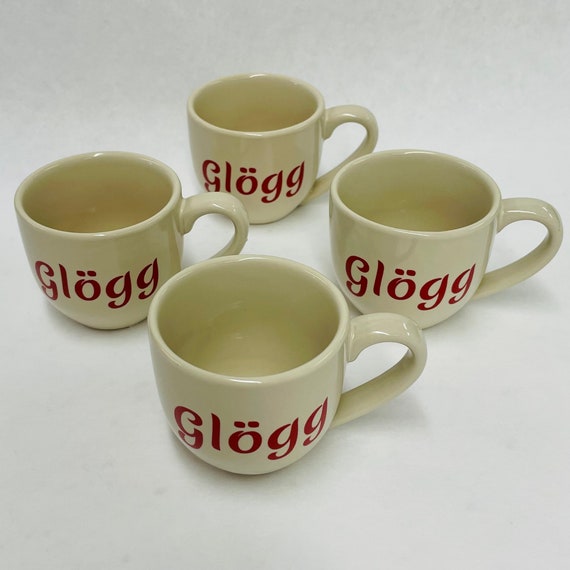This color photograph features a white table with four identical, empty coffee mugs arranged in a 2x2 grid. The mugs are a light beige or tan color with a slightly rounded bottom and medium-sized handles, all oriented to the right. Each mug has the word "GLOGG" inscribed on the front in dark red, lowercase lettering, with the 'O' adorned by two dots (ö). The interior of the mugs has a reddish tint, hinting that they may have contained something previously. The ceramic mugs have a shiny surface, indicating they have been fired, and the photograph allows a view from the front and slightly above, offering a glimpse inside each cup.